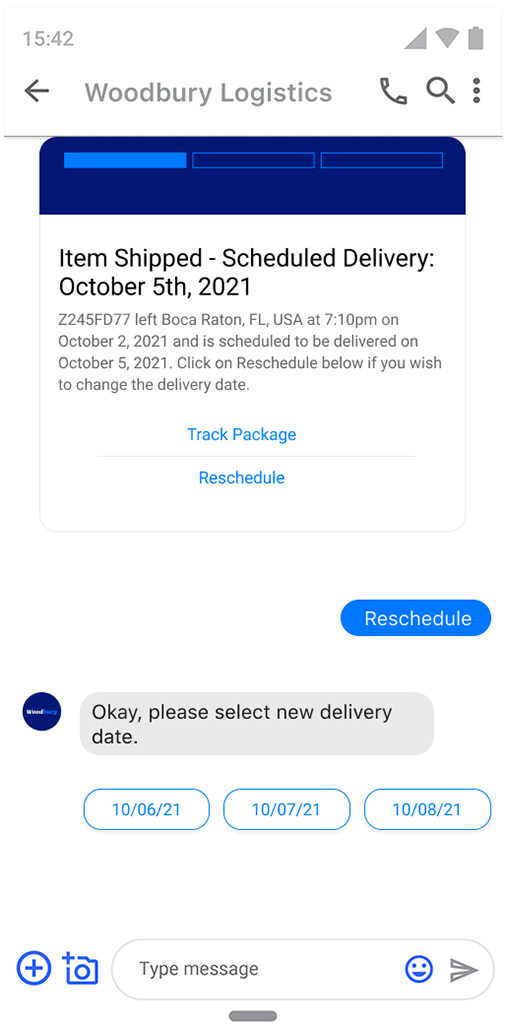A detailed screenshot captured from a mobile phone interface shows various elements against a white background. The top part of the screen displays the time "15:42" in gray text, indicating the use of the 24-hour time format. To the right, indicators for cell coverage, Wi-Fi, and battery status are visible. 

Below this, a black arrow pointing left is seen with the text "Woodbury Logistics" in gray beside it. Next to it are icons representing a black phone, a black magnifying glass, and three black buttons. Following this, there is a section with a dark blue background featuring lighter blue accents and shaded blue areas, creating a layered effect.

In the main white area, black text reads "Item Shipped," followed by a scheduled delivery date, "October 5th, 2021." Below this, light gray text shows the confirmation number, stating "Left USA at 07:10, October 7th, 2020," further reiterating the scheduled delivery on "October 5th, 2021." A prompt below invites users to "Click reschedule below if you wish to change the delivery date," followed by blue text options to "track package" or "reschedule." 

Towards the right, there's a blue button with white text saying "Rescheduled," accompanied by a logo that resembles the FedEx logo, featuring white and orange colors within a blue circle. Text in gray prompts the user to "Please select the new delivery date," followed by black text options for "10-6-21," "10-7-21," and "10-8-21." 

At the bottom right, there is a circle with a plus sign inside it, next to a camera icon, and a text input field labeled "type message" in black. Adjacent to this, a small blue smiley face and a black "send" button are visible. A grey bar is positioned at the very bottom center of the screen.